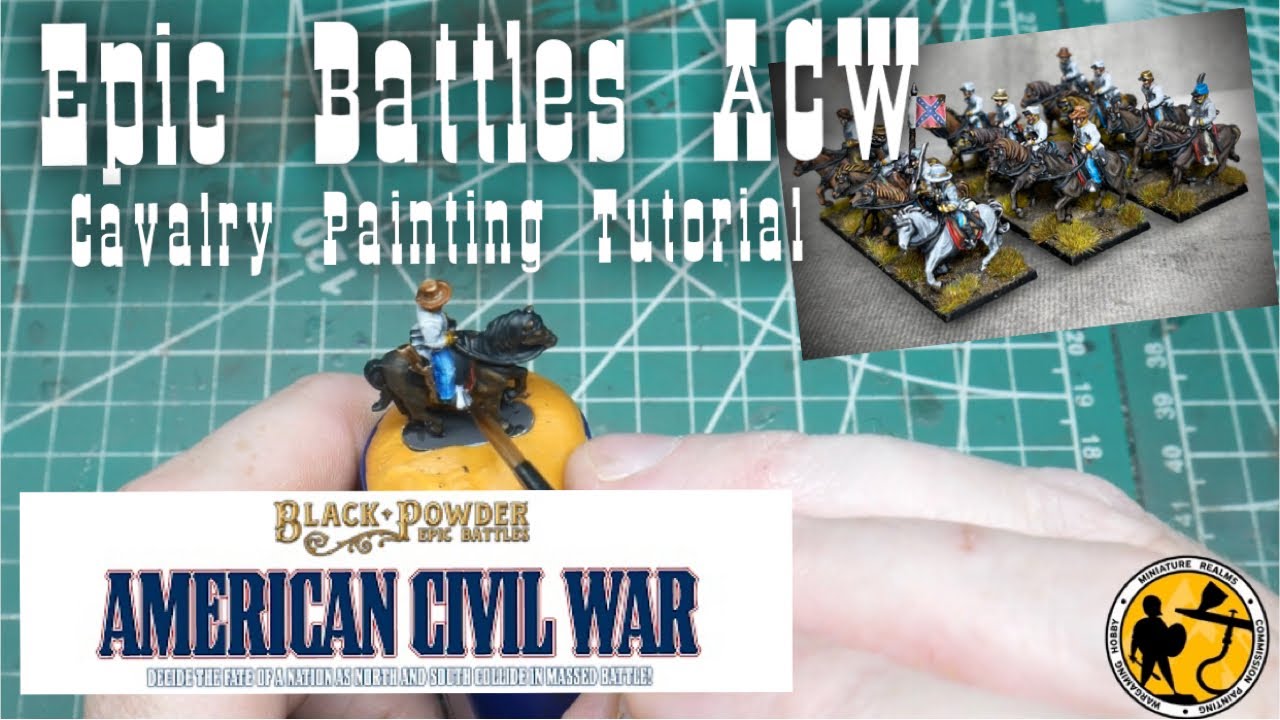The rectangular banner for the tutorial article or blog, twice as long in width as in height, is detailed and captivating. On the top left, large white text with a soft drop shadow reads "Epic Battles ACW Cavalry Painting Tutorial." This text overlays a close-up image of hands meticulously painting a cavalry figurine positioned on a round putty base, set against a crafting mat marked with white lines and numbers. The bottom left corner features a white rectangle with black text that announces, "Black Powder Epic Battles American Civil War." It continues with, "Decide the fate of a nation as North and South collide in massive battle!" Emphasizing the grand historical context of the figures being painted. On the top right, a small thumbnail showcases a completed cavalry army, one prominently wielding a Confederate flag, tying into the historical theme. The bottom right corner hosts a circular logo depicting the outline of a man with an airbrush, symbolizing the Painting War Coming Hobby. The overall detailed visual encapsulates the essence of a tutorial for painting intricate Civil War cavalry figurines, perfect for history and hobby enthusiasts alike.